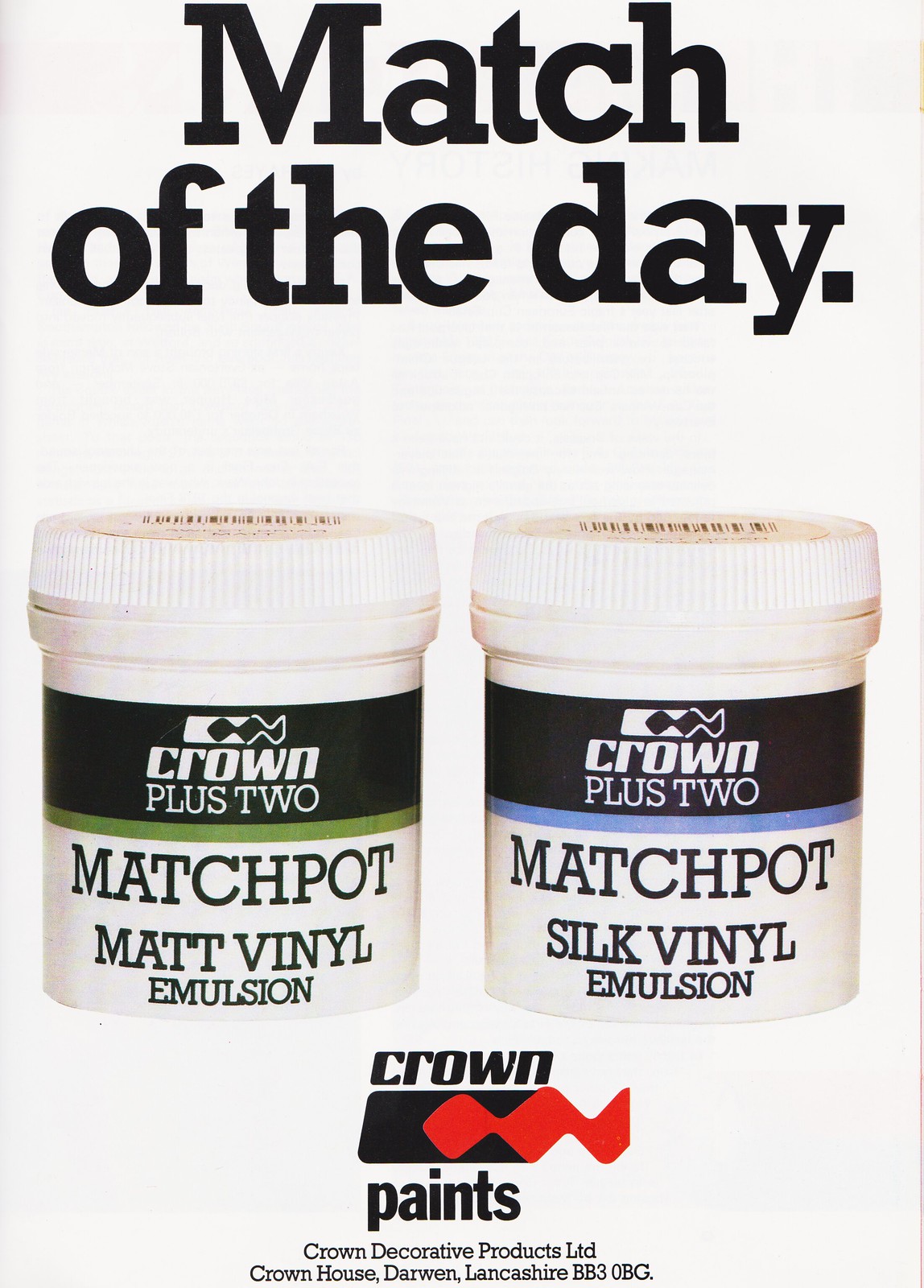The image is an advertisement titled "Match of the Day" with a black background and bold capitalized white letters at the top. It showcases two white plastic containers side by side. Both containers have the label "CROWN PLUS 2" against a black background. The container on the left features a blue stripe beneath the label and reads "Match Pot Silk Vinyl Emulsion," while the container on the right has a green stripe and states "Match Pot Matte Vinyl Emulsion." At the bottom, the advertisement bears the "Crown Paints" logo, which consists of a black rectangle with a red swirl. Below this logo, the text reads "Crown Decorative Products Ltd, Crown House, Darwen, Lancashire, BB3 OBG."